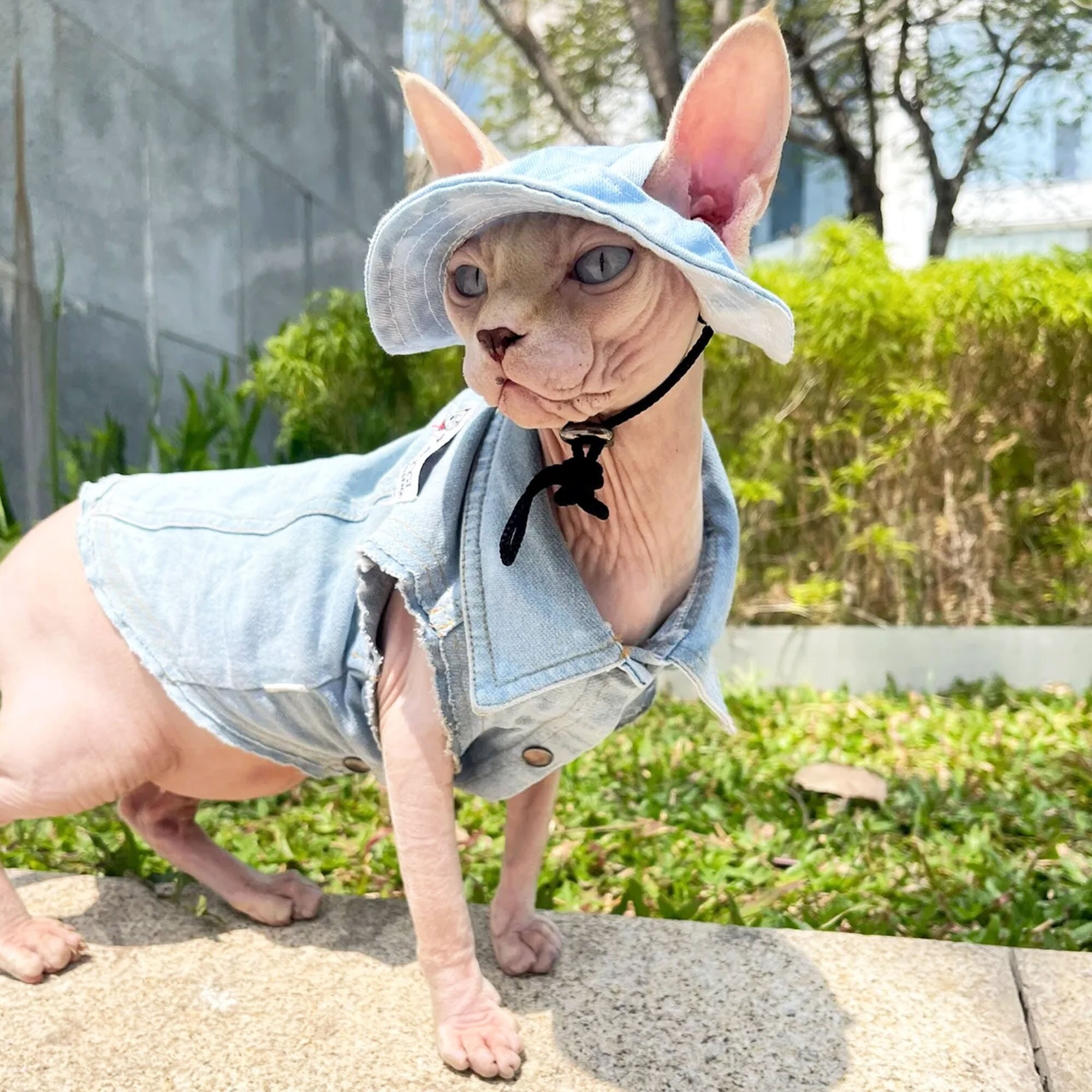This outdoor photograph captures a charming hairless Devon Rex cat with a delicate pink skin tone, sitting attentively on a concrete walkway. Its large, wrinkly ears peek out from a faded blue denim hat, which is tied under its chin with a black cord. The cat's striking blue eyes and darker-colored nose add to its unique appearance. Adorned in a light blue, buttoned-down denim jacket, the cat strikes a pose with its bare, petite legs visibly protruding through the armholes. Behind the cat, a lush backdrop of green grass, a garden, and a tall tree provide a natural contrast, while a marble or stone wall is visible to the left, and a light-colored large building stands in the distance. The photograph captures both the cat's endearing presence and the picturesque outdoor setting.